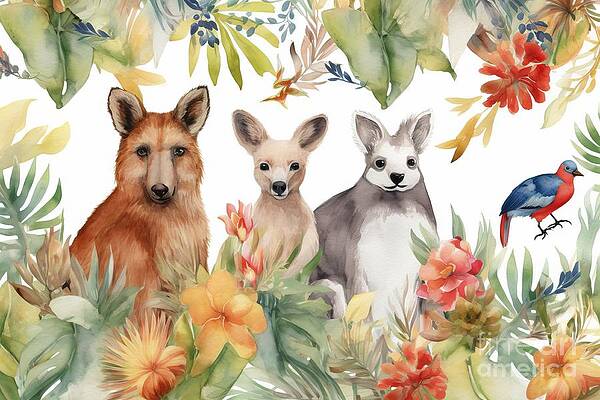The image, reminiscent of a children's picture book illustration, is a soft pastel, almost watercolor depiction of a lush tropical scene brimming with vibrant foliage and diverse flora. Four animals are aligned from left to right amid an array of tropical plants and flowers that range in colors from peach and light pink to dark red and blue. On the far left, there is a large brown bear with a black nose, eyes, and ears, exuding a peaceful demeanor. Beside the bear is what appears to be a kangaroo or a small deer, characterized by a tan body and similarly marked black facial features. The third animal, with large ears and a black and white fur pattern, could be a sloth-like creature or a rabbit, adding an element of curiosity to the scene. To the rightmost of the group is a striking bird, seemingly midair with a vivid red chest, blue wings, and a sharp pointy beak turned towards the east. The overall composition is charming and busy, with an intricate mix of pastel greens, oranges, and blues that enrich the tropical ambiance.